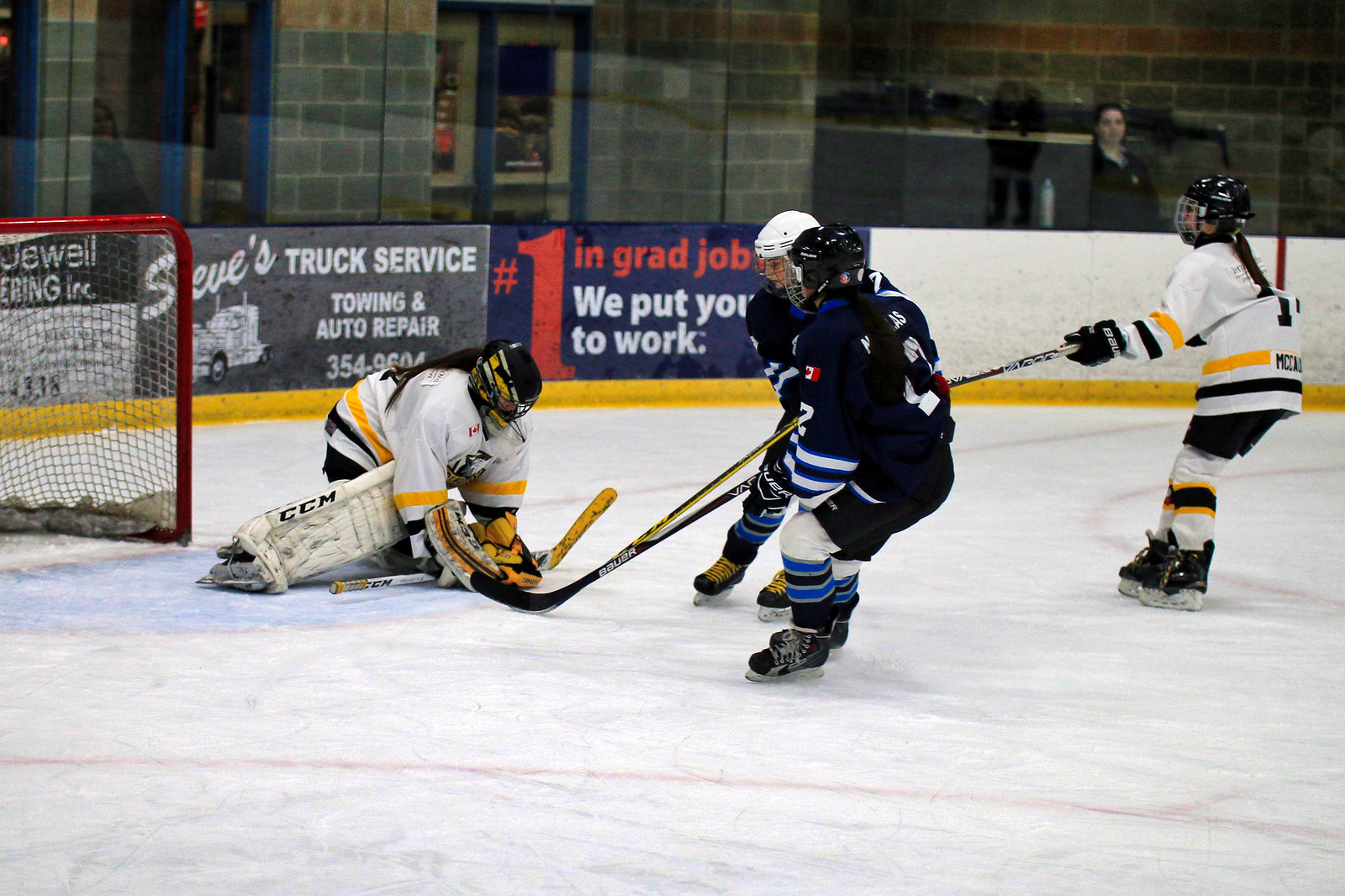The image captures a dynamic hockey game with players energetically skating on the rink. Two teams are competing, one dressed in black uniforms and the other in white and black uniforms. Four players are prominently seen in action, each with hockey sticks in hand, against the backdrop of a white ice surface. On the left side of the frame, a red goal post is visible. Behind the rink, the arena wall is adorned with various advertisements. Notably, one ad in the middle reads, "Number one in grad job. We put you to work," though parts of it are obscured. Another ad to the left says, "Steve's Truck Service, Towing and Auto Repair," along with the phone number 3549604 and a truck design. Two spectators can also be seen watching through the glass.